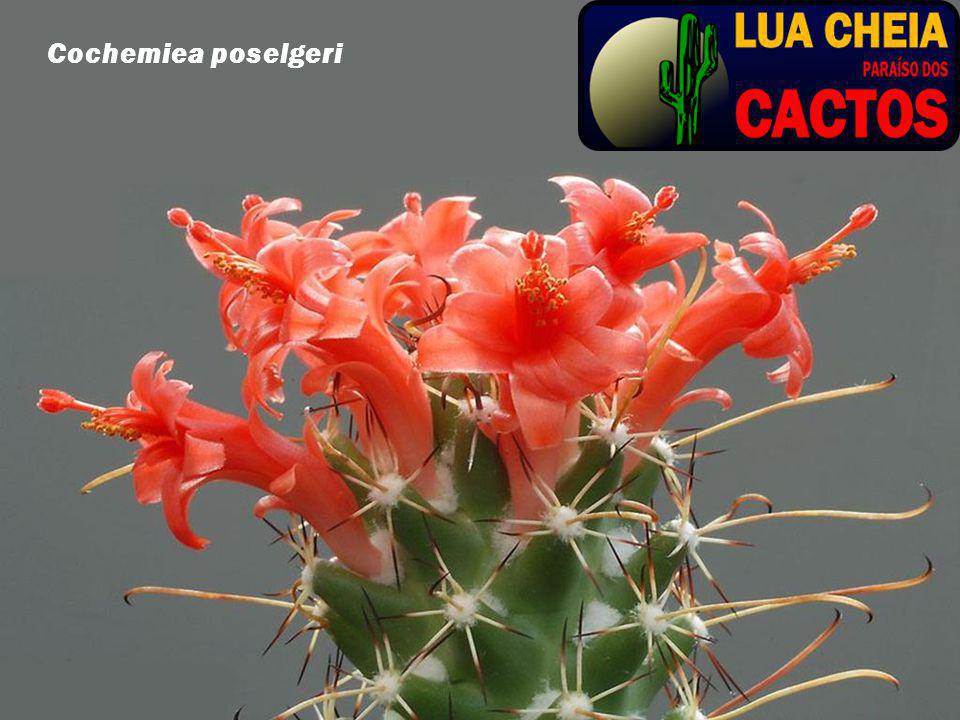The image features a close-up of a green cactus adorned with numerous white-tipped spikes, resembling small cotton balls at their base, and white toothpick-like thorns that are round-tipped. The cactus is blooming with striking reddish-pink flowers, their vibrant hue reminiscent of a flamingo. These flowers have little petals unfurled and delicate stems emerging from their centers. The background of the image is gray. In the upper left corner, the text "Cochenia postelgerii" appears in bold white font, suggesting a scientific name. The top right corner features a dark blue rectangular tab containing a logo with a full moon and a cartoon cactus. The text in this section reads "Lua Chia" in bold yellow font, with "Paraíso Dos" in smaller red font beneath it, followed by "Cactos" in larger font.